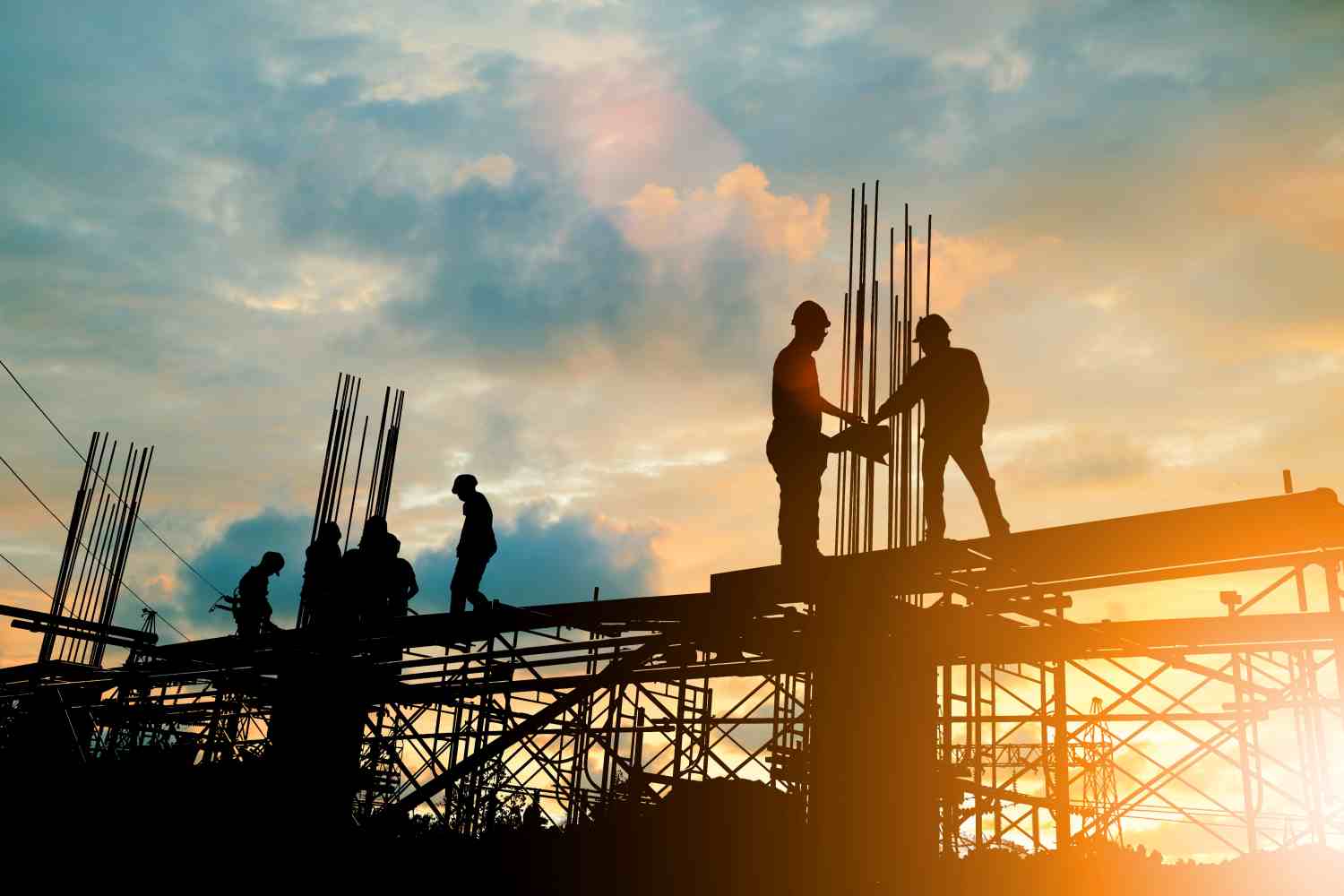In this evocative image of a construction site at sunset, the sky is a vibrant blend of blue, pink, and orange hues, accentuated by puffy clouds. Silhouetted against this stunning backdrop, several men, wearing hard hats and safety harnesses, diligently work on a metal structure. The two men on the right are closely observing a piece of equipment. Positioned on scaffolding, they are surrounded by vertical rebar, integral for cement pouring. On the left, a group of four or five men collaboratively engage in building tasks, supported by rods and pillars that frame the scaffolding below. The entire scene is bathed in the golden glow of the setting sun, casting long shadows and highlighting the construction efforts.